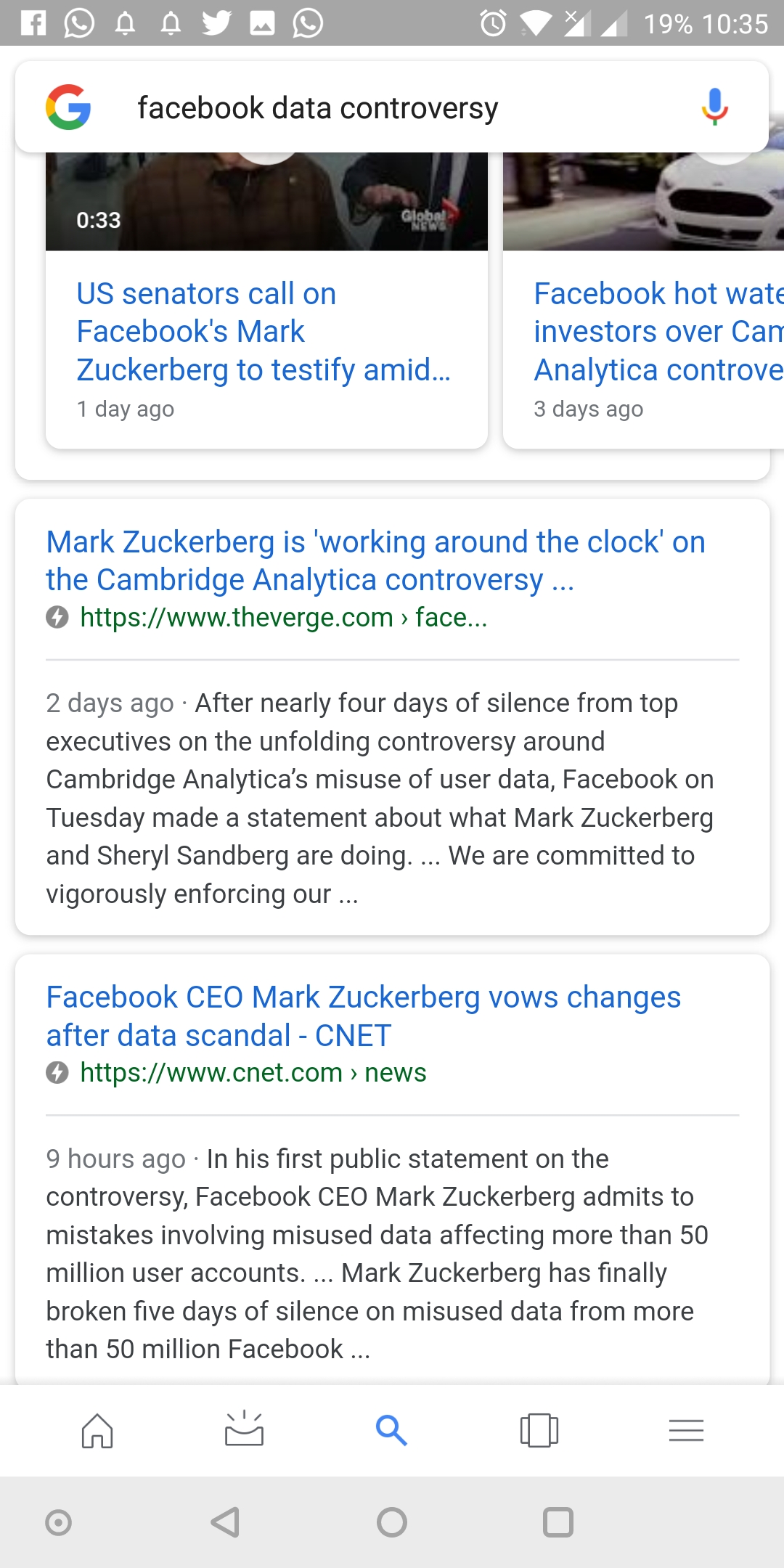This is a detailed screenshot of a Google search results page focused on the Facebook data controversy. The page displays four search results. 

The first two results are video links. The first video, titled "US Senator Calls on Facebook's Mark Zuckerberg to Testify," is 33 seconds long and was posted one day ago. The second video, titled "Facebook in Hot Water Over Analytical Controversy," features a thumbnail of a white car parked on a curb and was posted three days ago.

The third search result contains only text and states, "Mark Zuckerberg is working around the clock on the Cambridge Analytica controversy," originating from TheVerge.com and posted two days ago.

The fourth result is from CNET.com News, posted nine hours ago, and is titled "Facebook CEO Mark Zuckerberg Vows Changes After Data Scandal."

At the very top of the screenshot, a gray status bar includes several icons. The time displayed is 10:35, and the battery percentage is at 19%, located at the top right corner. The top left corner displays several icons including a Facebook icon, a call icon, two bell icons, a Twitter icon, a portrait icon, and another call icon. All of this is set against a white background.